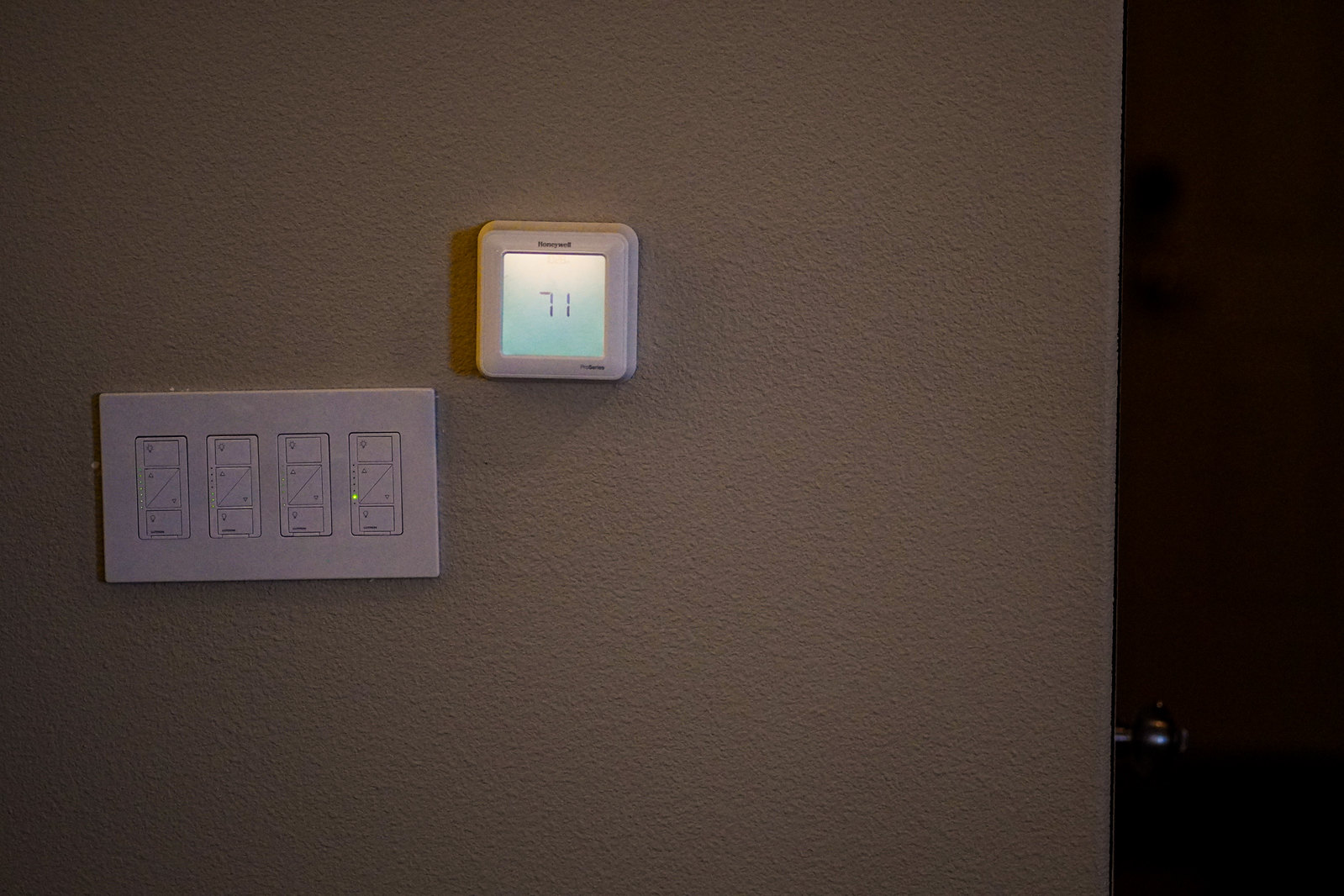The photograph captures a section of a living room wall in a house, featuring a textured stucco finish similar to a popcorn ceiling effect. Two distinct panels are visible. 

The first panel, located left of center and lower on the wall, is white with four vertical segments, each divided into three sections. Each segment includes small lights: the leftmost segment has six green lights, the next one three green lights, followed by one or two green lights in the third segment, and a single, brightest green light on the rightmost segment. The purpose of these buttons is not immediately clear.

In the center of the wall, there is a small, white square Honeywell thermostat set to 71 degrees Fahrenheit. The thermostat appears to feature a touch screen, displayed with a gradient effect transitioning from white to light blue.